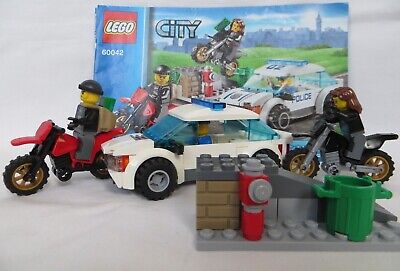This is a close-up photo of a constructed LEGO City set, specifically LEGO kit 60042. Dominating the scene is a thrilling chase scenario: a LEGO criminal, identifiable by his backpack stuffed with green money, zooms away on a red motorcycle. Hot on his tail is a sleek LEGO police car, a white vehicle with blue lights on top and black tires, driven by a police officer in a blue suit.

In addition to these primary characters, there is a LEGO figurine of a girl with long brown hair riding another motorcycle colored black and silver. The setting includes a concrete-like LEGO area featuring a brick wall, a red LEGO fire hydrant, and a green LEGO trash can. A sloped ramp-like structure evokes the image of a dynamic urban environment. 

In the background, the LEGO City kit box is visible, displaying vibrant artwork of the set that includes a police chase against a city skyline. The box art shows a police officer and a female motorcyclist chasing a criminal, complementing the built scene in the foreground.